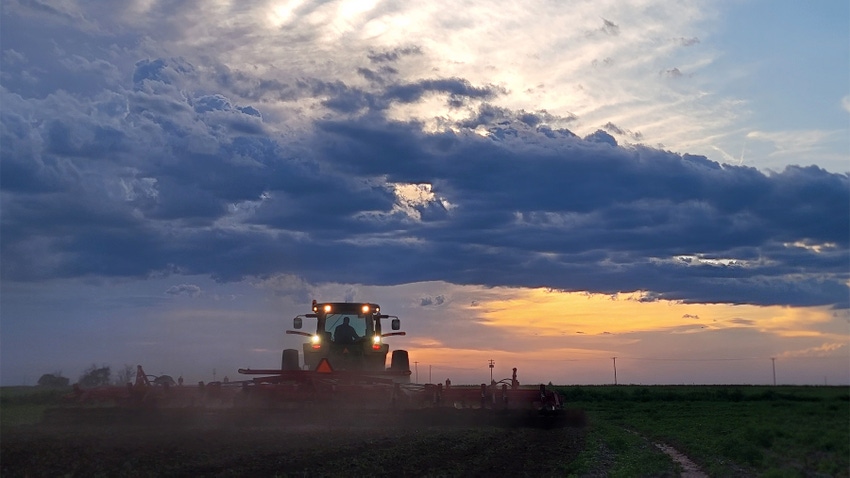The photograph captures a tranquil scene of a large combine harvester on an expansive field during the twilight of either sunset or sunrise. The combine harvester, illuminated with four bright lights, is facing towards the viewer with a slightly left-center position in the frame. The figure of a farmer is visible inside the cab, diligently maneuvering the harvester through the field. 

The sky above is a gradient of deep blues, grays, and patches of white clouds. The upper portion of the image showcases dark blue clouds stretching from the top left to the top right corner, with clearer blue skies still visible in the top right. Below this, the sky transitions to more gray tones, eventually blending into a soft, orange-yellow glow where the sun is either setting or rising. This glow delicately lights the bottom of the clouds and creates a dusky atmosphere, hinting at the day's end.

In the background, parallel rows of tall telephone poles can be seen extending into the distance on the right-hand side, adding depth to the scene. The field itself is dark green, appearing well-tilled and showing signs of previous planting. Dust kicked up by the harvester floats in the air, contributing to the overall imagery of a productive, bustling farm.

An orange triangle safety marker is prominently displayed on the back of the harvester, and the machinery is equipped with a wide blade being used to turn over the soil. This serene but industrious landscape photograph, presented in landscape orientation, beautifully captures the essence of farming life under the vast, colorful sky of either dawn or dusk.